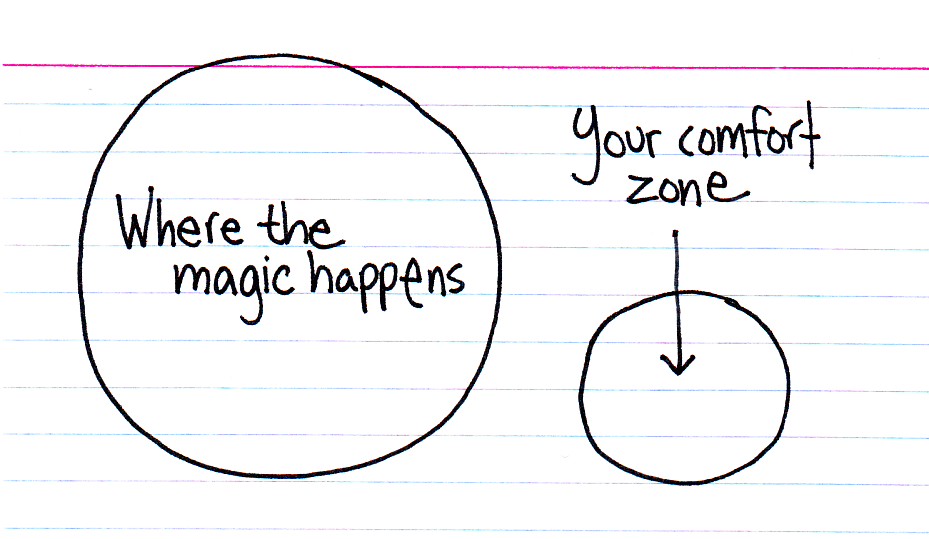This image features a detailed hand-drawn illustration created on lined paper. A nearly solid, bright pink line, likely drawn with a pencil and ruler, stretches horizontally across the top of the image. Overlaying the thin blue lines typical of lined paper, the pink line intersects slightly with a large, imperfect black circle, hand-drawn to the left side of the page. Written within this large circle in handwritten text is the phrase, "where the magic happens." Just outside this larger circle, towards the right, lies a smaller circle labeled "your comfort zone." An arrow is drawn from beneath the "your comfort zone" label pointing towards the inside of the smaller circle, suggesting a journey from the comfort zone to the area where "the magic happens." The illustration appears to convey a motivational message about stepping out of one's comfort zone to achieve extraordinary results.